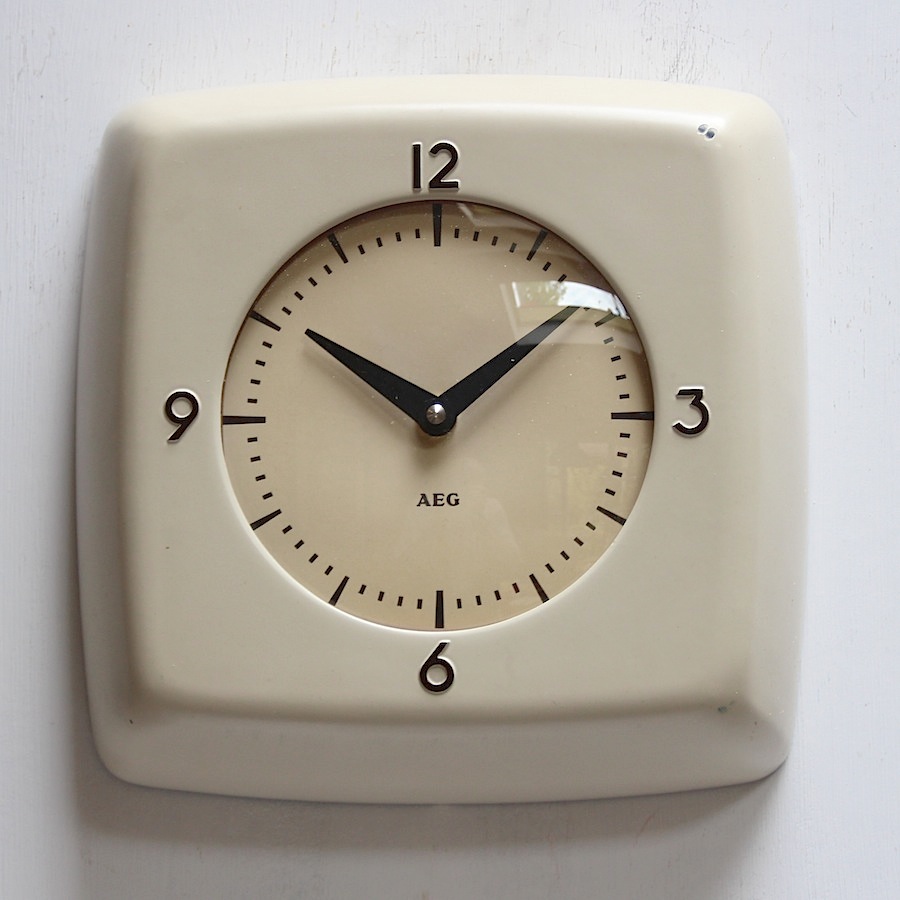A meticulously photographed vintage AEG clock is prominently displayed against a white-painted wooden wall. The clock, likely from the mid-century modern era, features a clean cream-colored face with minimalistic markers. Only the hours of 12, 3, 6, and 9 are numerically detailed, represented in a classic, understated font, while the remaining hours are denoted by simple slashes. Elegant hour and minute hands point to the precise time. In the reflective surface of the clock, one can discern the faint outlines of a nearby window, through which lush greenery or a cypress tree and a portion of the sky can be seen, adding an extra layer of depth and ambiance to the serene setting.